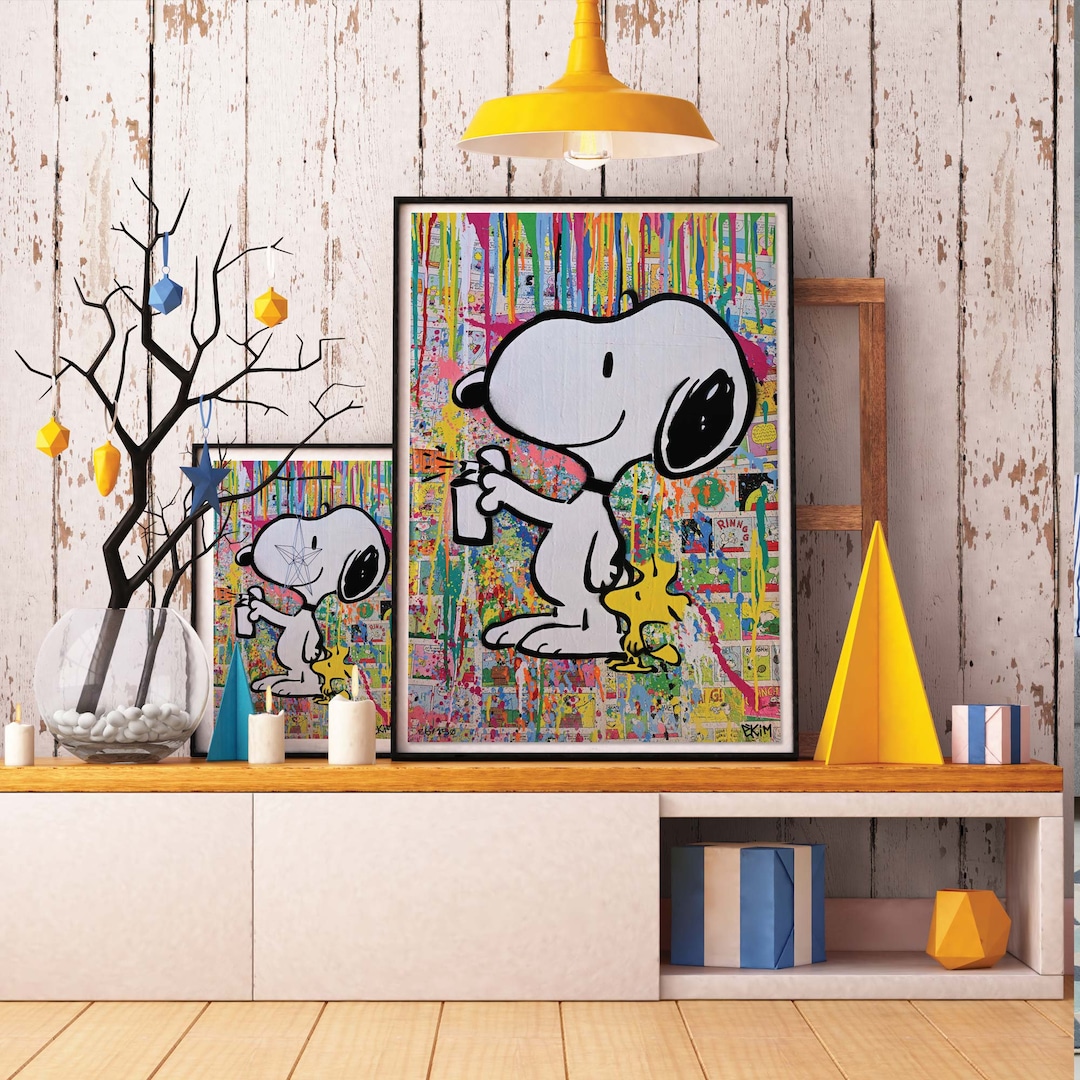The image shows a well-lit child's playroom with a blonde wood floor and a rustic white wooden background marked with faded and used spots. Dominating the scene is a low white cabinet with a wooden bench top, on which rests a large artistic poster of Snoopy and Woodstock against rainbow paint stripes, accompanied by a smaller duplicate image to its left. Centered above the display is a yellow lamp fixture with a translucent bulb.

To the left of the posters is a distinctive black tree branch adorned with yellow and blue ornaments, including star and polygon shapes, all contained within a fishbowl filled with white stone pebbles. Below the posters, a small blue and white striped box and yellow polygon cubes sit on shelves within the open cabinet. Further to the right is a striking yellow, 3D pyramid shape, adding to the room's coordinated blue and yellow color scheme. The entire setup exudes a playful yet artistically thoughtful atmosphere, perfect for a child's imaginative play.